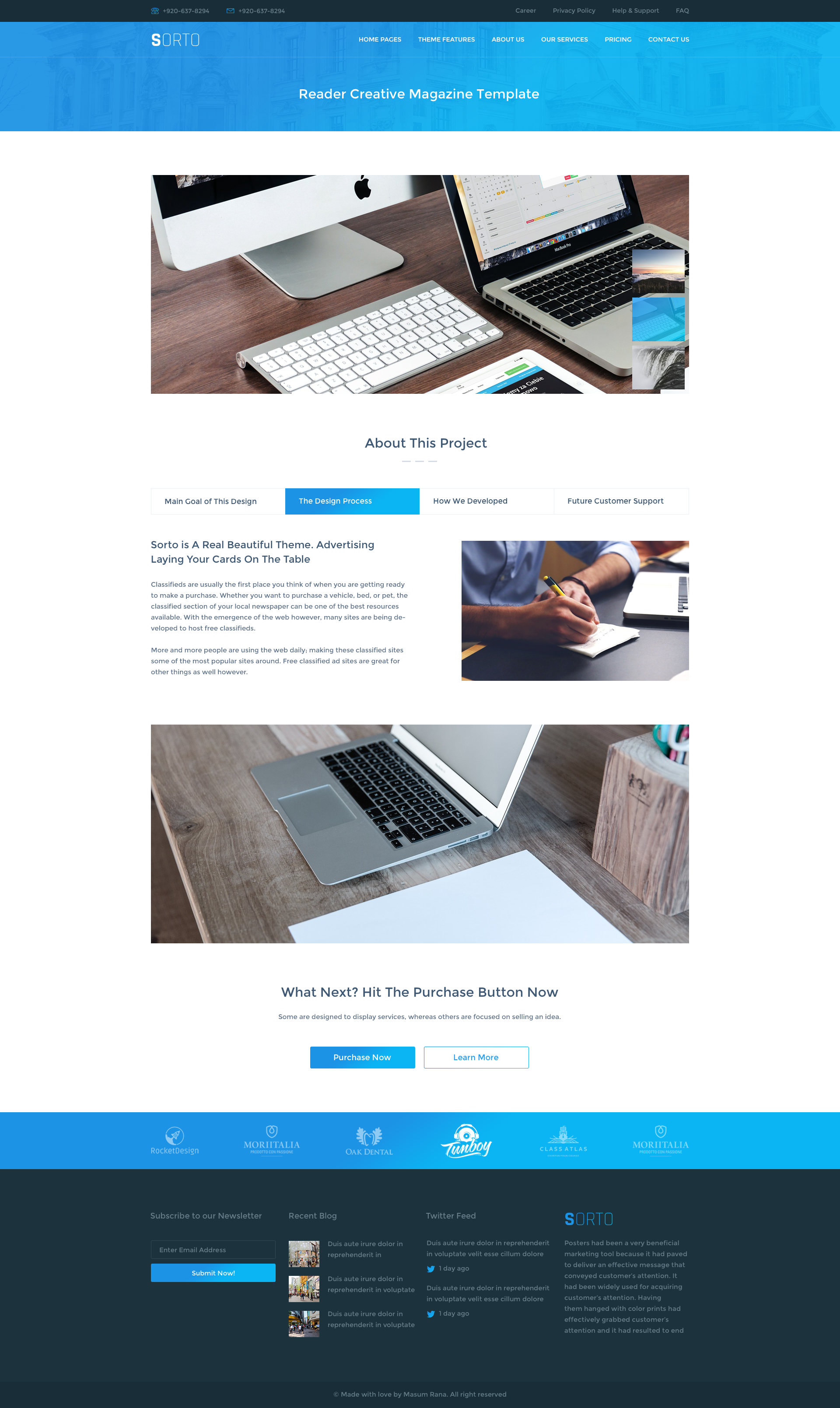**Screenshot Description: Design Template for a Creative Magazine Website**

The screenshot depicts a comprehensive layout of a website design template, specifically tailored for a creative magazine. At the top of the page, there is a blue header section. This section features a thin black bar running along the top, which includes several menu options aligned to the right. On the far left of the blue header, the word "SORTO" is prominently displayed in white.

Further details of the page include:

- **Header Section:**
  - **Logo:** Located on the top left within the light blue header.
  - **Menu Options:** Six white menu options are positioned on the right side of the header.

- **Main Content Area:**
  - **Header Image:** Below the blue header, a substantial header image showcases a workspace setup, including a laptop, an Apple monitor, and a keyboard.
  - **Project Introduction:** Directly below the header image, there is a prominent title stating "About This Project."
  - **Interactive Buttons:** Beneath the title are four buttons, with the second button highlighted in light blue, indicating an active or selected state.

- **Content Layout:**
  - **Text Column:** Positioned on the left side below the buttons, providing space for descriptive or informational text.
  - **Images:** 
    - An image situated on the right side adjacent to the text column.
    - Another image placed directly below the first image on the right side.

The layout is well-structured, balancing visual components with textual information, indicative of a user-friendly and visually appealing website design template aimed at creative magazine presentations.